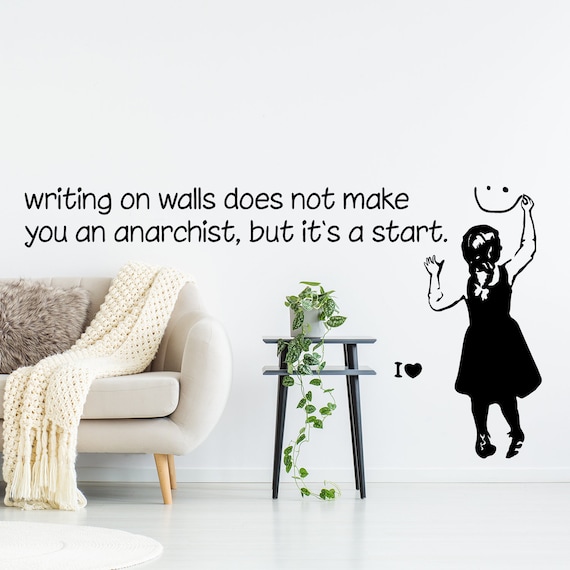The image depicts a minimalist living room with an all-white decor featuring white walls and white floors. To the left, there is a sophisticated white rounded couch standing on light wooden legs, adorned with a gray fluffy pillow and a white knitted blanket draped over the side. Adjacent to the couch, a dark side table holds a plant in a white planter, with leaves extending downwards, almost touching the floor. The focal point of the image, however, is the black writing on the central white wall that reads, "Writing on walls does not make you an anarchist, but it's a start." Below the text is a detailed black ink drawing of a little girl wearing a dress and finishing a smiley face sketch on the wall. Nearby, in black ink, are the words "I ❤️." This detailed interplay between the furniture and the artwork creates a thoughtful and artistic atmosphere typical of a stylish living room.